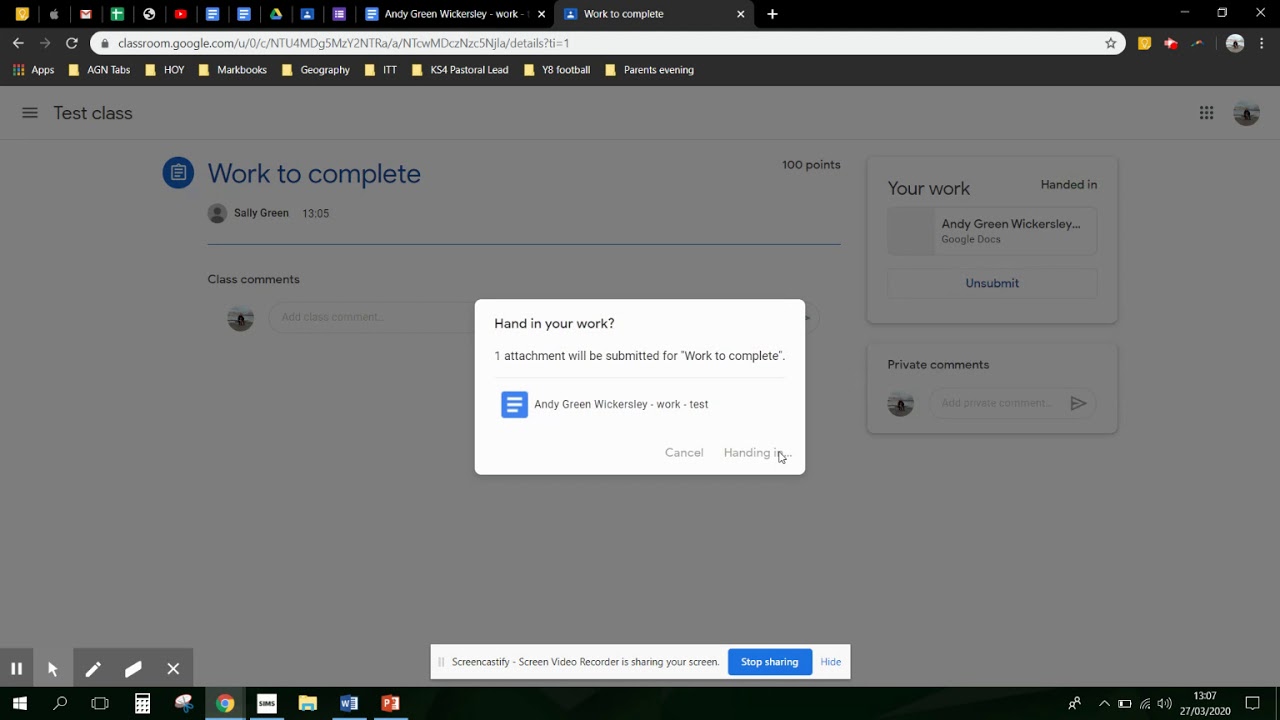The image showcases a typical interface of Google Classroom, visible through a browser with the URL classroom.google.com. The top section of the browser includes a dark theme with various symbols and bookmarked pages.

The main section of the browser displays a dark gray background with a prominent white rectangle at the center. This rectangle contains text in dark gray or light black, stating: "Hand in your work? One attachment will be submitted for Work to Complete." Below this text is a blue box with three horizontal bars, symbolizing a menu, labeled "Andy Green Wickersley Work Test." Further down, there are options to either "Cancel" or "Hand In."

Towards the bottom right corner of the screen, a cursor is present, and at the very bottom is an indication that "Screencastify Screen Video Recording is Sharing Your Screen," accompanied by a blue bar with the option to "Stop sharing" and another option in light blue labeled "Hide."

On the top left of the dark gray background, "Test Class" is labeled, and further right is a blue heading "Work to Complete," associated with "100 points" on the right side of the page. Under this heading, there is a small icon of a person within a circle, labeled "Sally Green," along with a timestamp and a section labeled "Class Comments."

To the right side of the page, there is a rectangle featuring text that reads "Your Work Handed In: Andy Green Wickersley Google Docs." Below this, there is a blue clickable symbol labeled "Unsubmit," followed by a section for "Private Comments" within a smaller box.